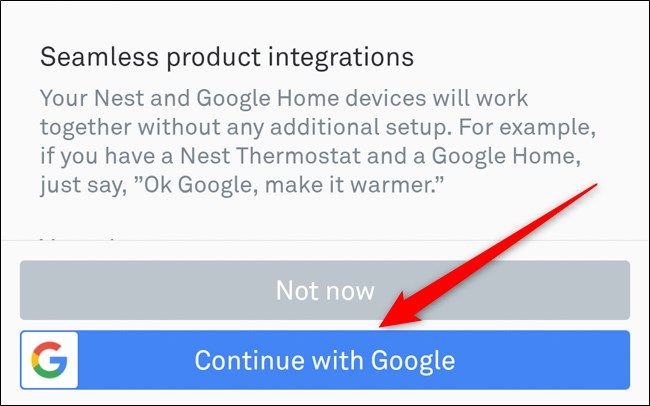The image resembles a user interface on a digital device, most likely a computer or a smartphone. It features a clean white background framed by a black rectangular outline. At the top of the rectangle, bold black text prominently displays the title: "Seamless product integrations." Directly beneath, smaller light gray text informs the user of the seamless integration between Nest and Google Home devices, stating: "Your Nest and Google Home devices will work together without any additional setup. For example, if you have a Nest thermostat and a Google Home, just say, 'OK, Google, make it warmer.'"

At the bottom of the rectangle, a wide gray bar stretches across the entire width, displaying the text "Not Now" in white. Below this, a more prominent blue bar also spans the rectangle's width. On the left side of this blue bar, a small white square contains the colorful Google 'G' logo. To the right of the logo, the blue bar continues with the text "Continue with Google" in white.

Additionally, a conspicuous red arrow starts from the middle right side of the image, pointing diagonally downward toward the "Continue with Google" button, seemingly guiding the user to click on it.